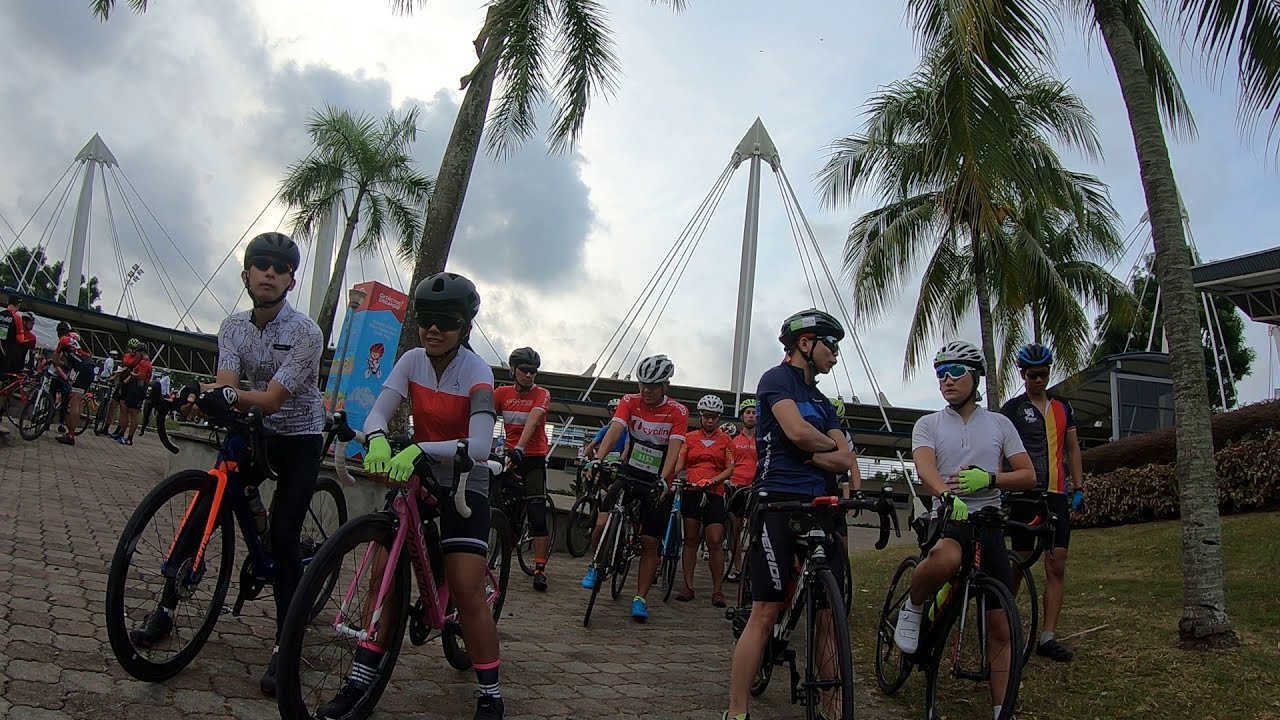This photograph captures a horizontally aligned rectangular image of a group of cyclists poised for a biking competition or race in what appears to be a park or public area. The cloudy sky is partly overcast with large puffy gray and white clouds concentrated more densely on the right side of the image. Tall palm trees punctuate the scene, with about ten prominently rising in the foreground.

Centered in the photo are several cyclists, all equipped with bike helmets and gloves in a variety of colors. In the front row, the riders sport diverse shirts—a white patterned shirt, a red and white shirt, a navy blue shirt, and a white shirt. Behind them, a section of the group uniformly dressed in red short sleeves stands out.

To the left, another cluster of mostly red-clad cyclists is visible, some standing next to their bikes. The participants, including an assortment of bright green and black gloves, appear ready and waiting for the race to begin, with a palpable sense of anticipation in the air.

In the background, large metal structures with triangular shapes and wires add an industrial touch to the otherwise natural landscape, and patches of grass and bushes peek out from the right side of the photograph. The cobblestone pathways and the overall gathering of cyclists and spectators hint at an organized event filled with enthusiasm and competitive spirit.